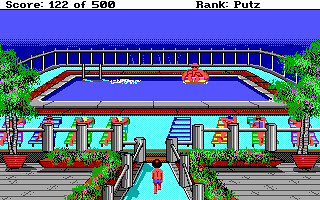In this vibrant screenshot from a video game, we can see the game's interface displaying a score of 122 out of 500 at the top. To the right of the score, the rank is indicated, although it says "rank puts," suggesting a placeholder or unconfigured text. The background features a serene blue, which could represent either a sky or the ocean, providing a tranquil setting. 

Central to the scene is an animated environment depicting a stylish pool area surrounded by a railing. To the left, there's a large, muscular or overweight character with a pinkish-red hue, striking a noticeable contrast against the serene backdrop. Alongside the pool, lounging chairs are arranged in a relaxed manner. Additionally, to the right, a character in light green attire is seen walking down an aisle towards the pool, adding a dynamic element to the scene. The overall atmosphere is lively and colorful, indicating a playful and engaging game environment.